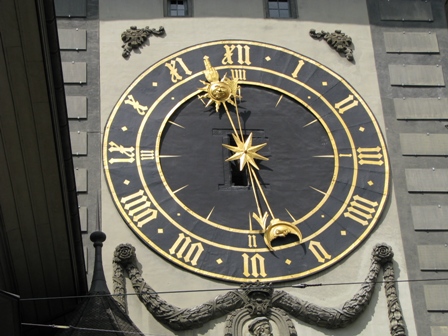This rectangular, landscape photo is a close-up shot of a large, ornate clock affixed to the façade of a stately gray building. The clock face is striking in black, complemented by gold numerals and hands. Intricately designed, one end of the clock's hand features a sun, while the other end showcases a half moon, with a star positioned at the center of the dial. The building itself is primarily gray, with darker gray elements adding to its grandeur. At the top of the structure, two windows are visible, along with a partial view of a black roof extending to the left, enhancing the architectural character captured in this image.